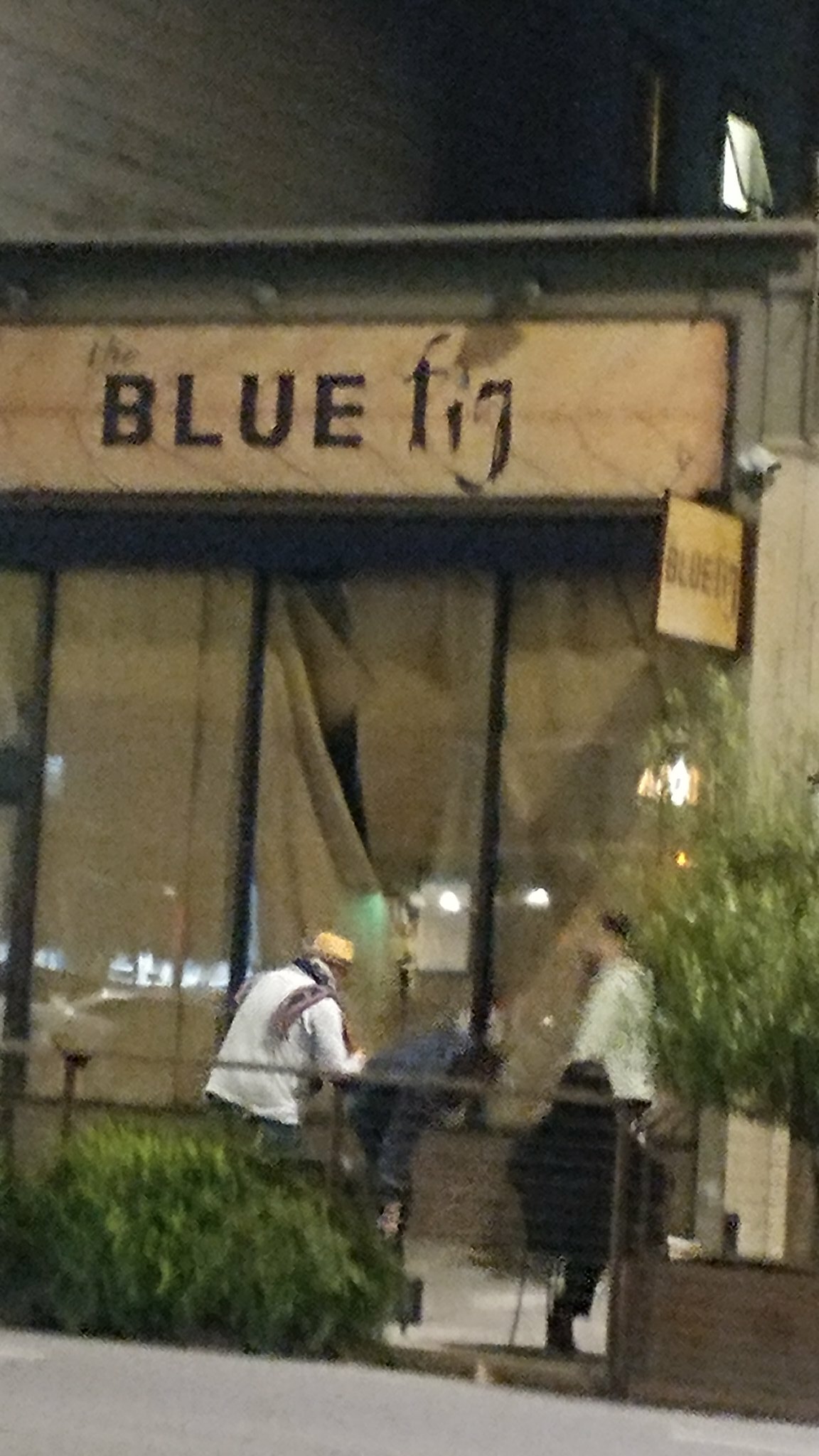The image depicts a scene on a stone-paved ground where lush greenery frames both sides with bushes, specifically located at the bottom left and right corners. A sturdy metal railing runs through the middle of the scene. At the top, a sign prominently reads "The Blue Fig," conveying the name of the establishment. Adjacent to this sign, it's reiterated with another "Blue Fig" sign, creating a sense of brand consistency.

The central focus is a large, reflective glass window, segmented by sleek black metal dividers. The windows are meticulously covered with a thin layer of brown paper, lending an air of mystery as they mask the interior while subtly allowing the night’s ambiance to seep through.

In the foreground, a person dressed in a white shirt and a distinctive yellow hat, along with a scarf draped around their neck resembling a snake, captures attention. To the right of this individual, another person is casually seated on a bench, adding a human element to this vibrant, night-time urban snapshot.